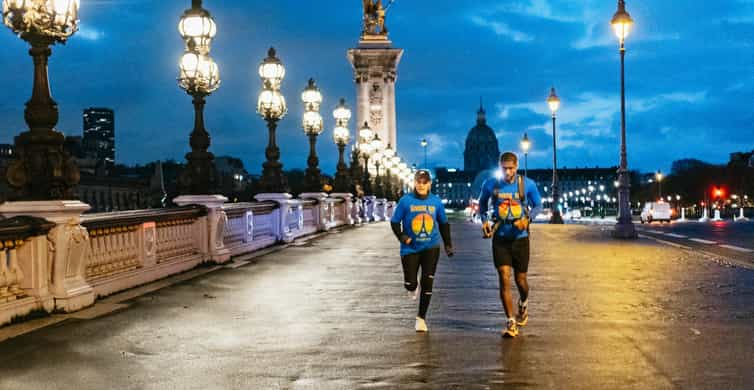In the foreground of this captivating twilight cityscape, a man and a woman, dressed in matching blue t-shirts adorned with a rainbow-colored Eiffel Tower insignia, command the scene as they run towards the camera. The man's outfit includes black shorts, black leggings with white strips around the knees, and brown-and-white sneakers, while the woman complements him with black long-sleeve attire underneath her t-shirt and crisp white sneakers. Both are mid-stride on a wide, well-lit pedestrian pathway, lined with elegant white lampposts, that could either be a bridge or a promenade flanking a busy street. Beyond the runners, the city's evening ambiance is punctuated by the distant glow of car headlights and streetlamps, suggesting an active thoroughfare. The backdrop showcases an impressive array of structures, including a discernible dome structure reminiscent of the U.S. Capitol Building, towering buildings, and statues, blending the architectural aesthetics of Washington, D.C., with a damp sidewalk illuminated by city lights.